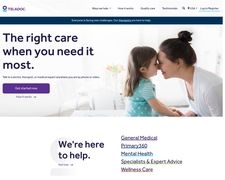The image depicts a webpage with low resolution, which blurs the text and elements when zoomed in, making them hard to read. At the top of the page, there is a navigation bar with the website's name, though the blurriness obscures the details. The background of this section is white with black text.

Beneath the navigation bar, there is a dark green strip with white text centered in it, reading "The right care when you need it most." Below this, unreadable text is present along with a purple button featuring white text, also unreadable.

To the right, there is a photograph capturing a touching moment between a white woman with dark hair styled in a bun and a young girl with dark brown hair. The woman's forehead is gently pressed against the girl's forehead. The girl wears a green shirt adorned with polka dots, while the woman is dressed in a white shirt. The background behind them is predominantly white with some indistinct variations.

Below the photograph, the website states, "We're here to help." Underneath, it includes the phrase "general medical" surrounded by other unreadable text, spread over five lines. The colors visible throughout the image include blue, green, purple, white, gray, and black.